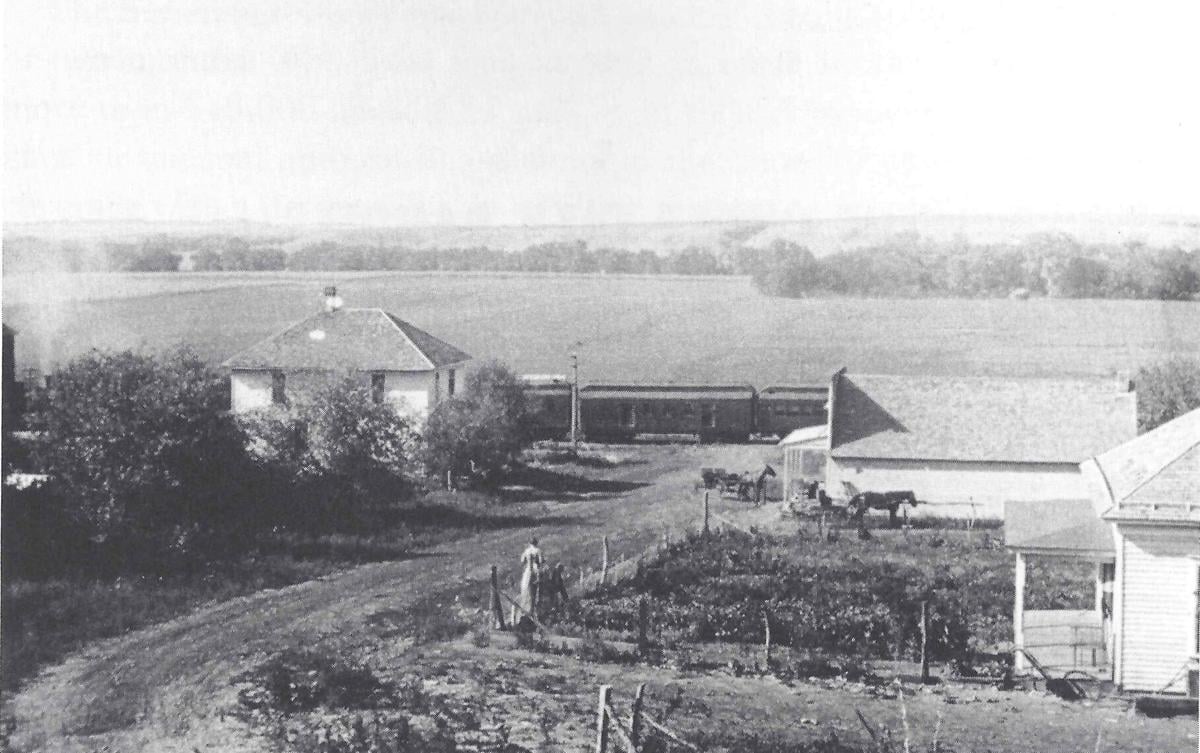This is a detailed black-and-white photograph, likely from the 1800s, capturing a serene, rural landscape. Prominently, the image features a modest wooden house, situated on the lower right corner, with multiple horses nearby. Centered in the photograph, a train with several cars is visibly passing by, hinting at either a nearby train station or a casual transit through the farmland. Behind the train, expansive grasslands stretch out, eventually blending into a line of distant trees that border the setting. A closer inspection reveals a person, possibly a woman, standing near a dirt road adjacent to the house. The sky appears predominantly white with subtle shades of gray. This scene, which might be from the American Midwest, reflects the simplicity and tranquility of country life in the 1800s.